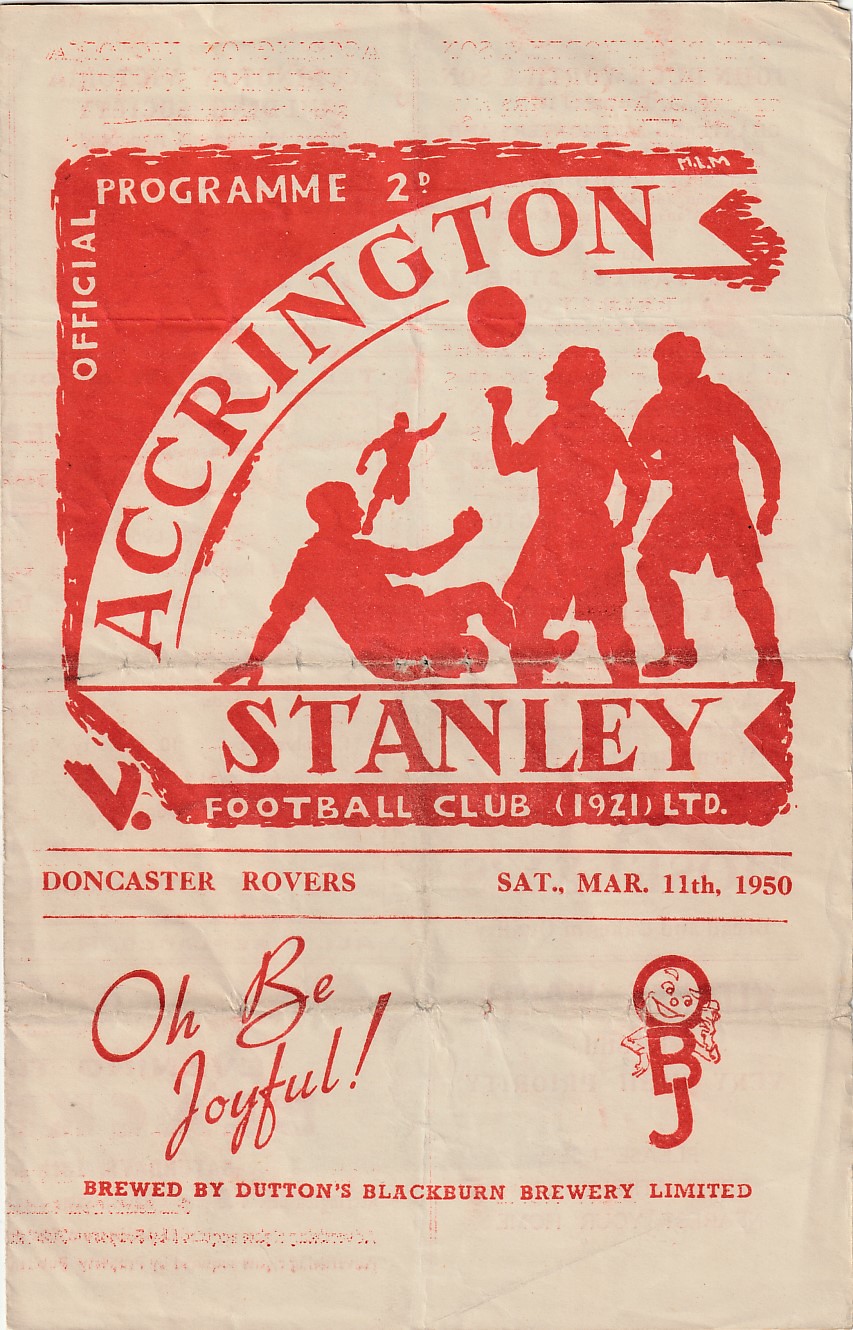The cover of this old soccer program, printed on slightly tanned white paper in red ink, features a collection of red silhouettes that vividly depict a soccer scene. At the top, there is a box with a red splotchy border containing the text "Official Program 2D." The word "Accrington" arcs prominently across the center in all caps, forming an elegant right angle with the word "Official" and the adjacent "Program" text positioned sideways. 

Below, the scene captures four soccer players in action: one sliding on the ground, another preparing to head the ball, a third in a defensive stance, and a fourth running towards them. Beneath these dynamic silhouettes, the text reads "Stanley Football Club 1921 Limited." 

A thin red line divides the lower section, which details the match information: "Doncaster Rovers, Saturday, March 11, 1950." At the bottom-left, "OB Joyful" is written in a festive cursive font, while to the right, "OBJ" is displayed within a whimsical logo featuring a cartoon face inside the O and small arms extending from the B and O. Below this, it states, "Brewed by Dutton's Blackbird Brewery Limited," indicating that OBJ is a style of beer.